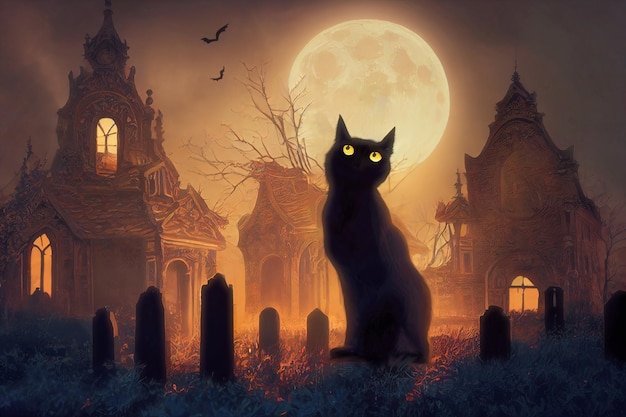This animated illustration captures a spooky Halloween night scene. Central to the image is the black silhouette of a cat with striking yellow eyes, looking up to the left. The cat stands in a cemetery, surrounded by headstones on both sides. The background features three large, dilapidated buildings with glowing orange windows, which give off an eerie, abandoned vibe. Above the cat, a full moon shines brightly, casting a yellowish-brown glow across the scene, and silhouetted bats fly in the foggy, grey sky. Dead trees with branch-like shapes and patches of dead grass further enhance the haunted atmosphere, with an orange light radiating from the ground behind the cat, adding to the overall eerie setting.